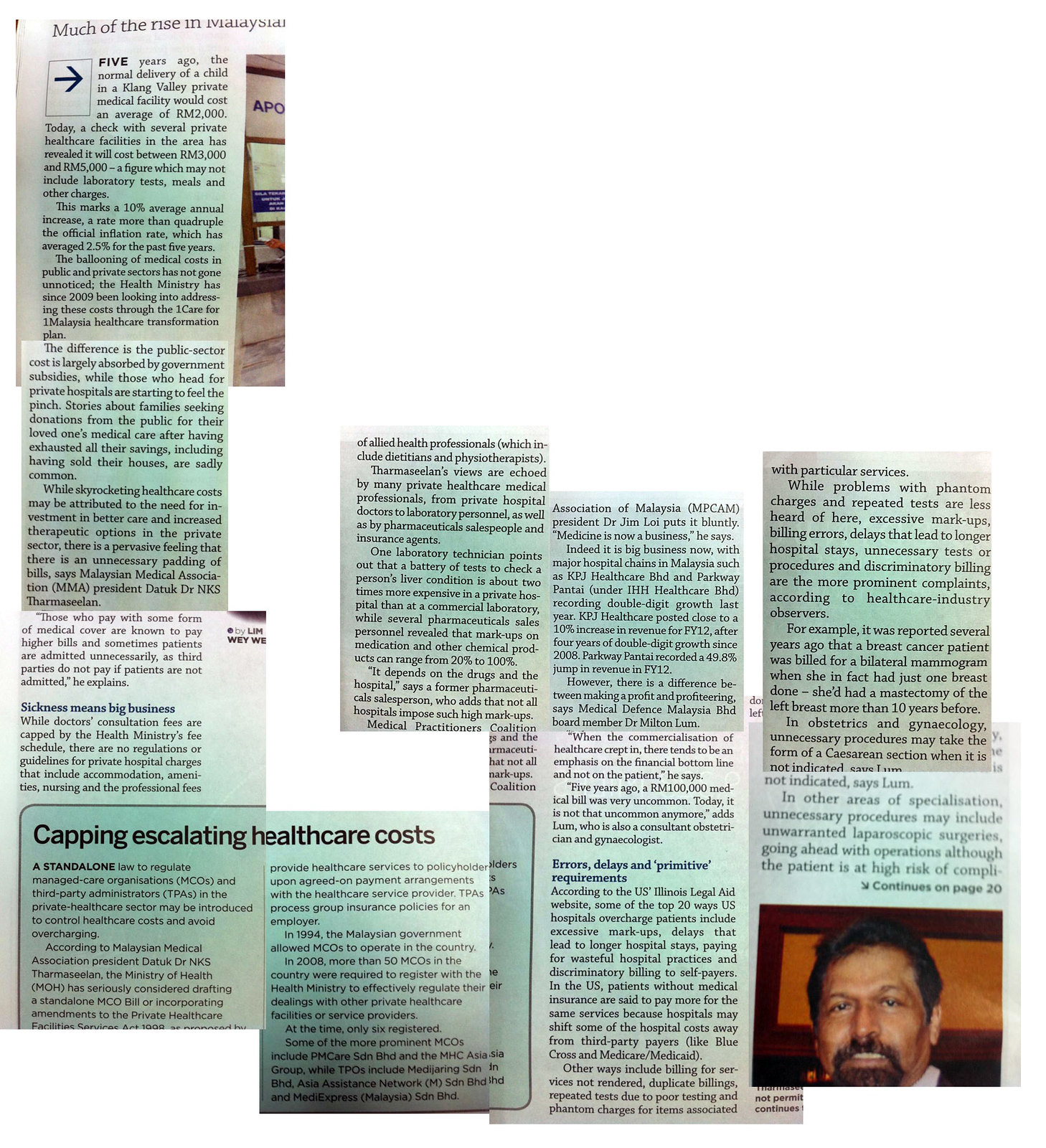This image is of a carefully arranged newspaper article that has been cut into long vertical strips and staggered on a white background with a subtle blue tint. The article focuses extensively on healthcare costs, particularly those associated with the Malaysian healthcare system, and includes discussions on escalating healthcare expenses. Notably, there's mention of regulatory measures to manage these costs, such as a proposed standalone law to oversee managed care organizations (MCOs) and third-party administrators (TPAs) in the private sector, aiming to prevent overcharging and billing errors. Towards the bottom left of the arrangement, there's a callout captioned “capping escalating healthcare costs.” In the lower right corner, there's a headshot of a Caucasian man with dark brown hair, a full mustache, and a goatee beard. The man's attire is not visible in the image. The article critiques unfair billing practices, delays, errors, and other issues that contribute to high healthcare costs and affect patients adversely.